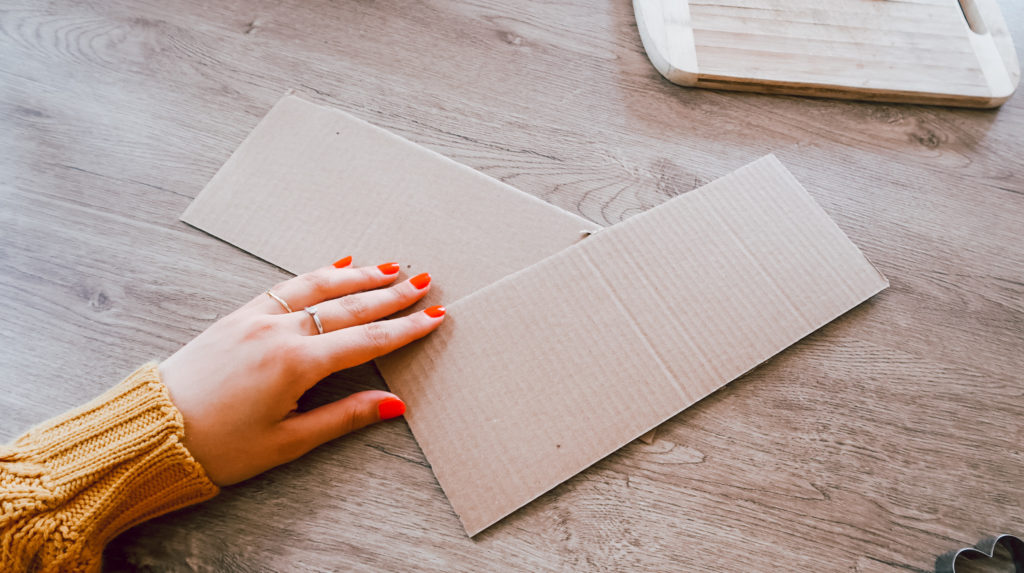In the image, a wooden table with distinct left-to-right wood grain pattern hosts a variety of objects and activities. At the center, a white Caucasian person, identifiable by their red-painted fingernails and adorned with two rings, is wearing an orange sweater, particularly visible on the left arm. To the bottom right of the frame, a small gray metal heart rests on the table's surface. Above it, two overlapping square cardboard pieces are positioned as if they are being adjusted or arranged by the person. Near the top of the table lies a wooden cutting board, characterized by rounded edges and a groove along its right side, with a darker line running through its middle. The arrangement suggests that the person might be preparing to cut or assemble something, potentially utilizing the metal heart and cardboard pieces.